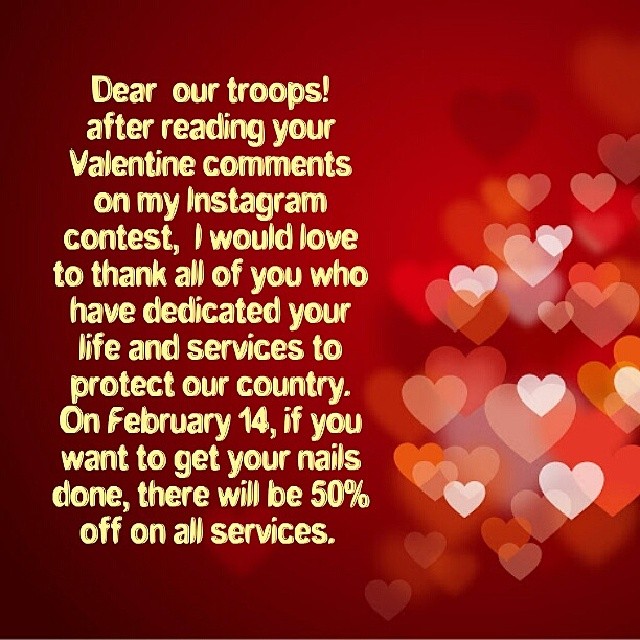The square image has a primarily red gradient background, transitioning from a bright red at the top right to a darker red at the bottom left. On the right-hand side of the image, there is an array of slightly opaque cartoon hearts in various shades, ranging from white, light pink, and dark pink to bright red and dark red. The left-hand side features a message in light yellow font that reads: "Dear Our Troops! After reading your Valentine comments on my Instagram contest, I would love to thank all of you who have dedicated your life and services to protect our country. On February 14th, if you want to get your nails done, there will be 50% off on all services." The overall design is vibrant and eye-catching, with the heartfelt message prominently displayed alongside the colorful hearts.